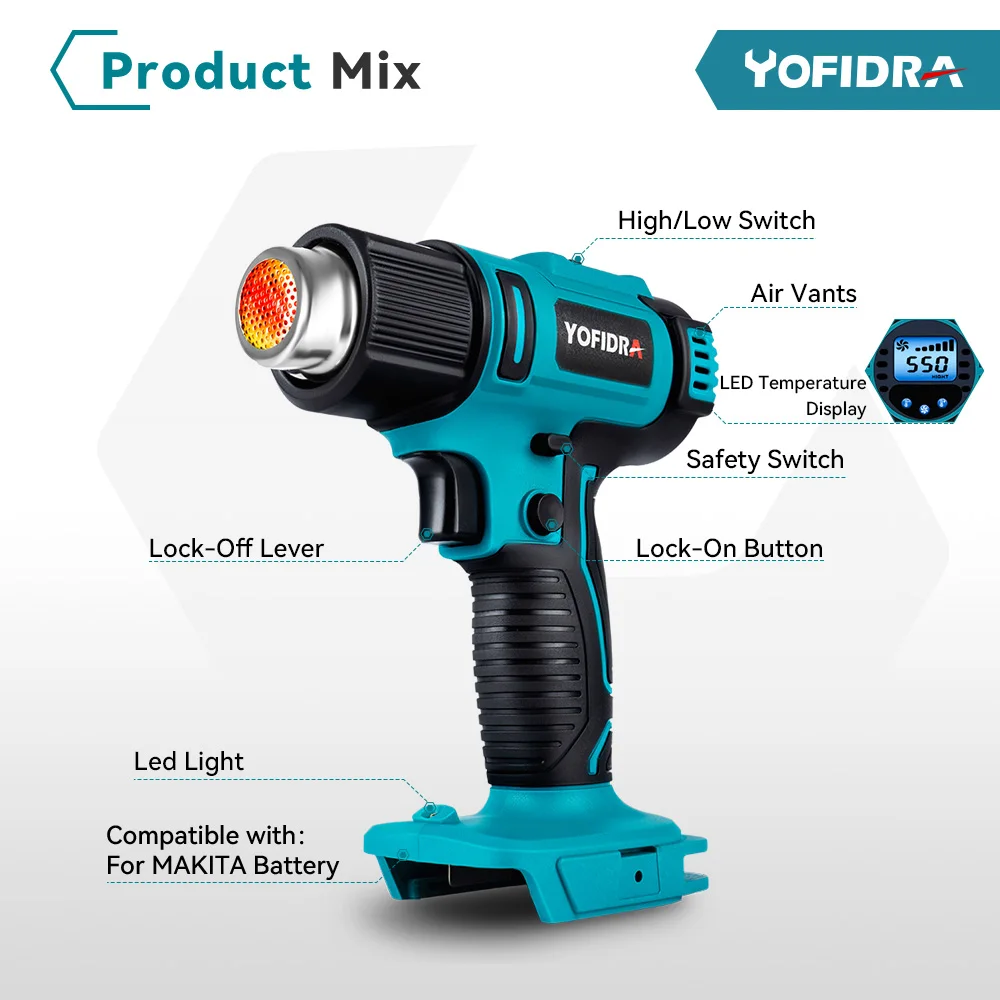This detailed photograph serves as an advertisement for a teal and black cordless power drill, extensively labeled to highlight its various features. The image features numerous text labels pinpointing different parts of the drill, such as the high/low switch, lock-on button, and lock-on lever. At the top of the image, the words "Product Mix" are displayed in teal and black text, respectively, with a teal banner in the top right corner bearing the brand name "Yofidra." Notably, the letter "Y" in Yofidra is depicted as a white wrench, adding a creative touch. The drill itself has a predominantly teal body with black accents, including the grip, buttons, and front section. The photograph employs blue dotted lines and black text to provide detailed descriptions of the drill's components and functions, ensuring that viewers are well-informed about the product's capabilities. Additionally, a portion of the background features an image of a blue and black temperature gauge, further emphasizing the brand’s diverse range of tools.